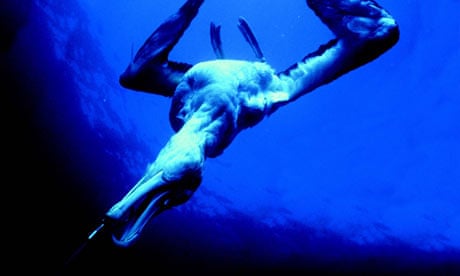The image captures an underwater scene with a striking contrast between different shades of blue and black. The right side of the picture is a lighter blue, fading to a darker blue towards the left and bottom sides, which form a curved L-shape in black, suggesting depth and perhaps indicating the ocean floor or shadows. In the center of this aquatic setting is a bird, likely a seagull, that appears upside down with its head submerged in the water, hunting for a small fish. The bird's webbed feet are visible in the upper middle part of the image, while its open beak points towards the lower left. Its wings are splayed out to the sides, creating an impression of it diving or being caught mid-motion, with the overall effect enhanced by the play of light filtering through the water.